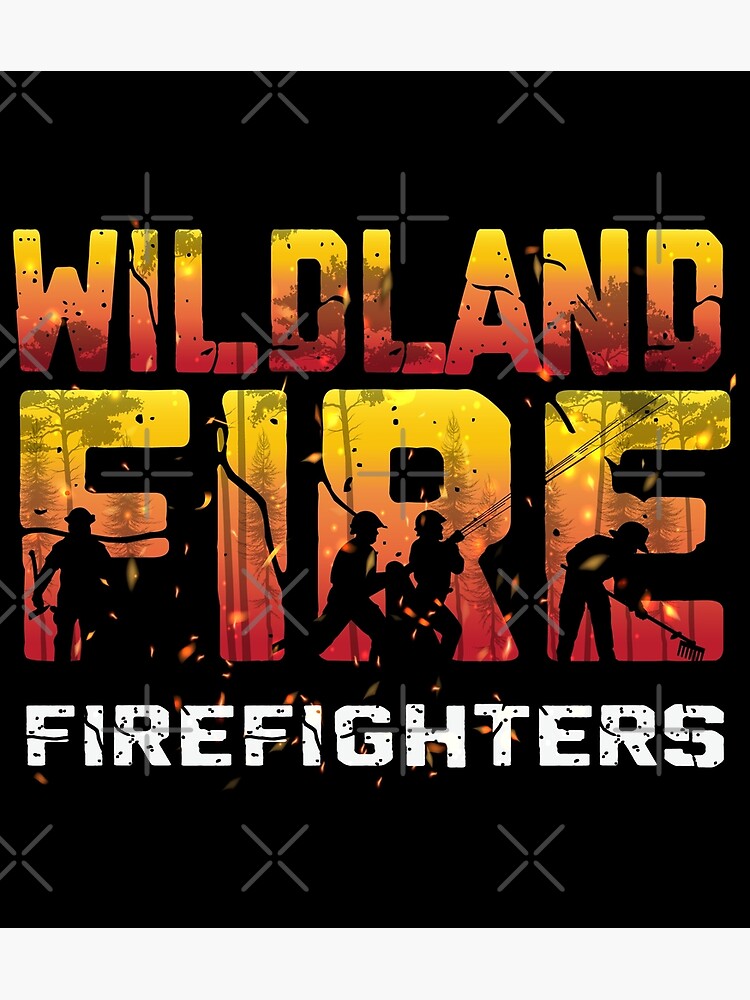This image is an intense depiction of wildland firefighters battling a forest blaze, characterized by the word "Wildland Fire" prominently displayed in a bold gradient font that transitions from yellow at the top to orange in the middle and red at the bottom. The word "fire" stands out, with each letter cut out from a photograph of the active fire scene. Within these letters, four firefighters are silhouetted against the flames — one on the right bent with a rake, two in the middle (one running and the other standing with a fire hose), and one on the left holding an axe. Behind them, trees and embers are visible, enhancing the dramatic effect.

The image's backdrop is solid black, accentuated by gray crosshairs and X shapes running across the image, adding a tactical aesthetic. Embers and ash seem to float across the entire picture, creating a dynamic and chaotic scene. The text "Firefighters" in white stands prominently against the dark background. The overall composition, with its vivid colors, silhouettes, and detailed environmental elements, effectively captures the peril and intensity of fighting wildland fires.